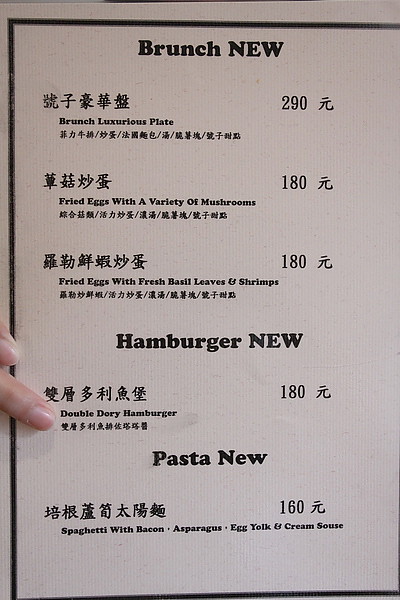This photo showcases a detailed menu printed on white paper with a black border and black lettering. At the top, the menu prominently displays the word "BRUNCH" followed by "NEW" in all caps. Directly below are Asian characters, accompanied by the English phrase "BRUNCH LUXURIOUS PLATE." Further down, more Asian characters follow, as well as a listed price of $2.90 next to an Asian currency symbol.

The menu introduces two additional new entrees. The first is described in English as "FRIED EGGS WITH A VARIETY OF MUSHROOMS," priced at $1.80, accompanied by Asian characters. The second entree reads, again in English, "FRIED EGGS WITH FRESH BASIL LEAVES AND SHRIMPS," also priced at $1.80, with corresponding Asian characters.

Further down, the menu features the word "HAMBURGER," followed by "NEW" in bold, all caps. The highlighted dish here is "DOUBLE DORY HAMBURGER," priced at $1.80, with surrounding Asian characters. A photograph embedded in the menu depicts fingers, likely from the person holding it, who appears to have feminine, natural nails.

At the bottom, under the heading "PASTA," the word "NEW" is written in regular typing. The pasta dish is described as "SPAGHETTI WITH BACON, ASPARAGUS, EGG YOLK AND CREAM SAUCE," listed for $1.60.